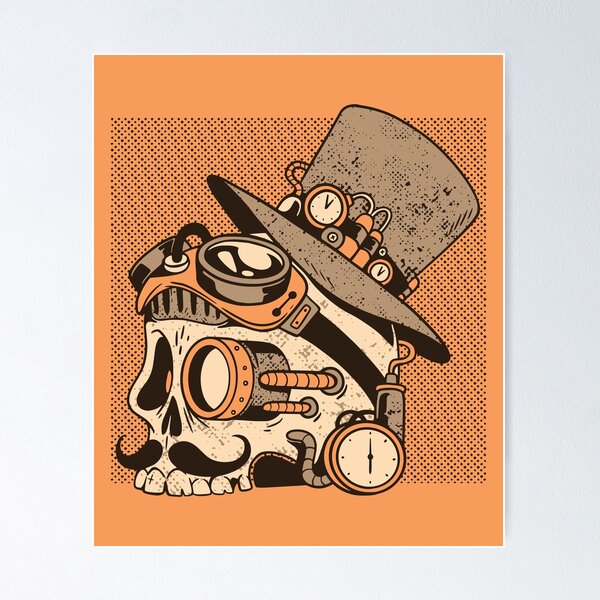This detailed art print features a visually striking steampunk-style illustration of a human skull, set against a primarily grayish-white background. The skull, with its top teeth intact, wears a tilted gray top hat adorned with small bombs or gas tanks wired around the hat band. Additionally, multiple watches or timers, resembling a bomb setup, are strategically placed on the hat and near where the ears would be.

The skull sports a black handlebar mustache and a monocle in one eye, adding to its unique character. A pair of rounded aviator glasses rests atop its forehead, with straps seemingly encircling the skull. The lower jaw is missing, enhancing the macabre aesthetic.

The artwork incorporates black-and-white illustration elements with a vibrant orange backdrop, bordered by hints of a white frame. The background behind the skull features a square pattern of tiny black dots, contributing texture and depth to the piece. The entire composition is printed on orange paper, heightening its visual impact and emphasizing the steampunk theme.